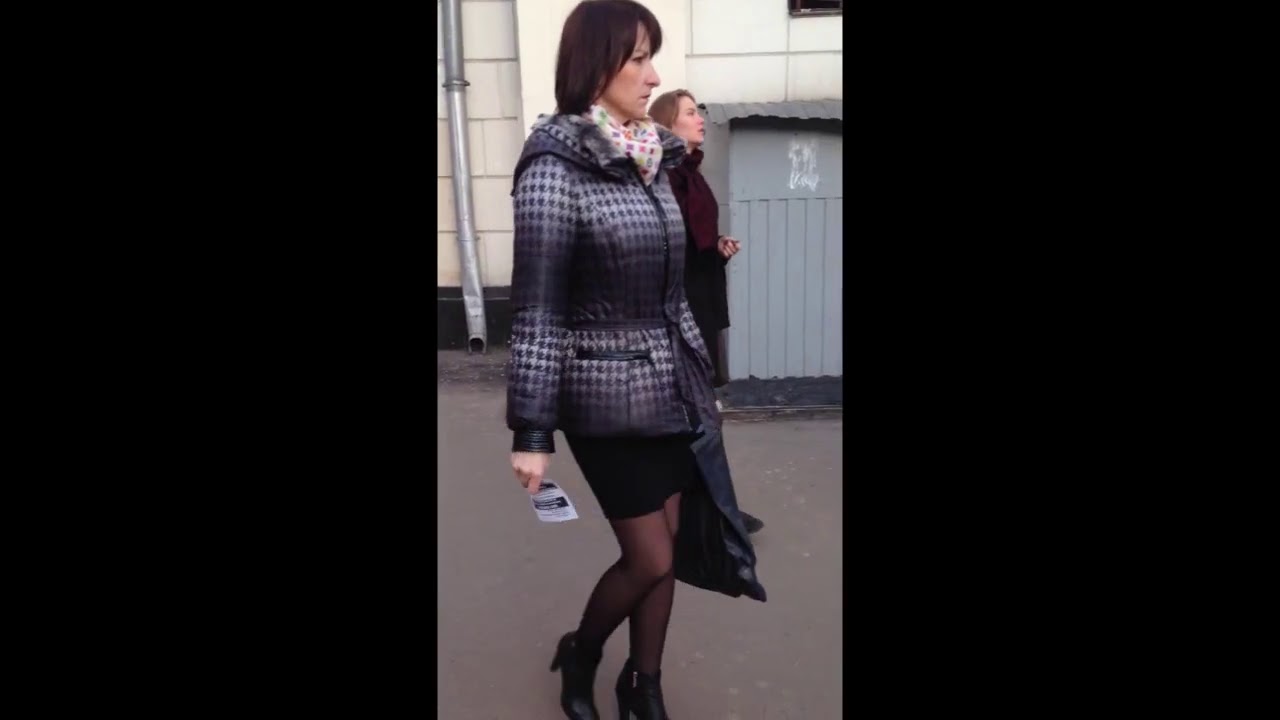In this photograph, two women are depicted standing in front of a white building with a gray portion visible on the right and a prominent drain spout running down from the upper left of the image. The woman in the foreground dominates the image. She has short brunette hair and a stern expression as she looks towards the right. She is clad in a distinctive houndstooth patterned jacket over a white and multicolored cravat, complemented by a black skirt, black hosiery, and black ankle boots. She holds a piece of paper in her right hand and appears to be carrying a shopping bag in her left hand. Behind her, another woman is shown in side profile, revealing the right side of her face. She wears a burgundy or maroon coat and has lighter brown hair. She is looking slightly upwards. Both women are presumably in a city setting, captured against a backdrop of an industrial-style building constructed of white concrete blocks with a visible metal pipe extending from the roof. The scene is framed with wide black borders on either side, lending a sense of focus and containment to the image.